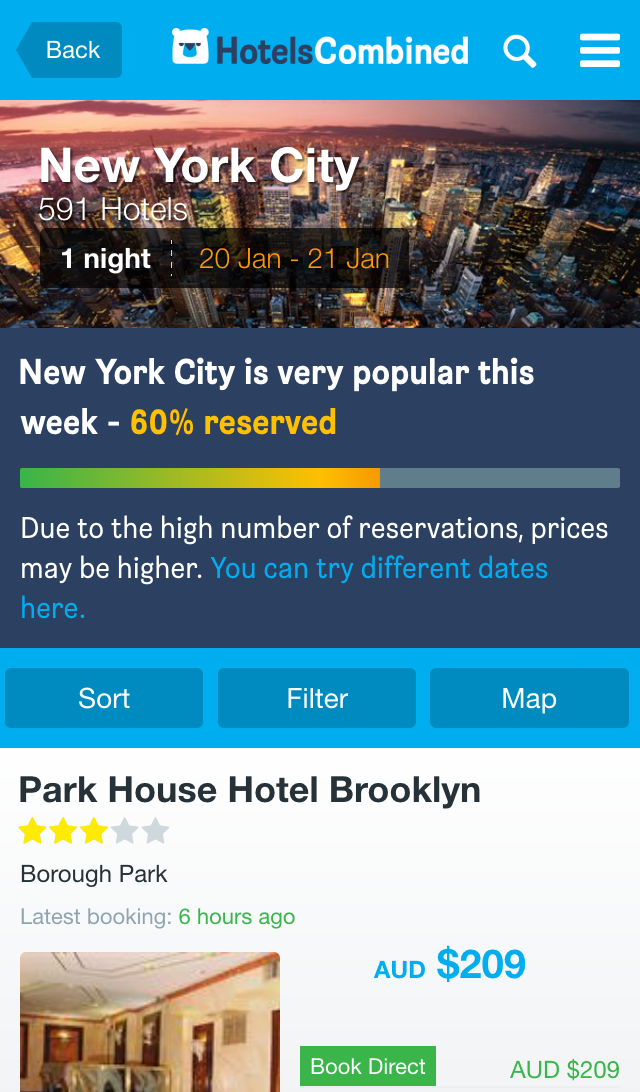The image is a screenshot taken from a mobile device displaying a Hotels Combined app interface. 

At the top of the screen is a horizontal light blue bar, which houses a gray back button labeled "back" in white text. The bar prominently features the Hotels Combined logo, consisting of a white bear head with a blue snout to the left of the words "Hotels Combined." The word "Hotels" is in black, while "Combined" is in white. Immediately to the right of the logo is a search icon.

Beneath the header, the screen showcases a photograph of New York City's skyline dominated by its iconic skyscrapers. Superimposed on this image, white text reads, "New York City, 591 Hotels, One Night." An orange text below specifies the dates "20 January to 21 January."

Further down, additional white text mentions, "New York City is very popular this week, 60% reserved," emphasizing the demand with "60% reserved" again in white.